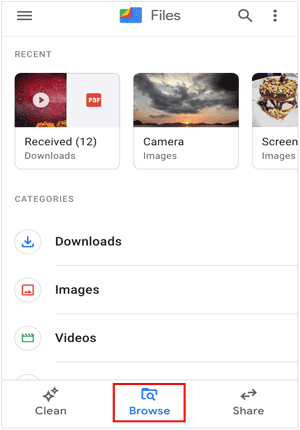In the detailed image presented, the focal point is a blue square. Positioned in the upper left corner of this square are three vibrant colors—green, yellow, and red—accompanying the word "Files." Directly below, the word "Recent" is visible. Adjacent to this area is a clickable box featuring a play arrow icon, with a red background. Below this element, the text "Received (12) Downloads" is displayed. 

To the side, a picturesque image of the sky during the late evening captures the setting sun amidst dark gray clouds. Underneath this evocative scene, the words "Camera" and "Images" are noted. Further to the right, "Screen Images" is depicted, showing what appears to be a gold crown. Various categories are outlined, including "Downloads," "Images," and "Videos."

At the very bottom left corner, the word "Clean" is positioned with two four-sided star symbols situated above it. Enclosed in a red box is the word "Browse," rendered in blue text, accompanied by an icon of a folder with a magnifying glass. Lastly, in gray text, the word "Share" appears with small arrows pointing left and right situated above it.